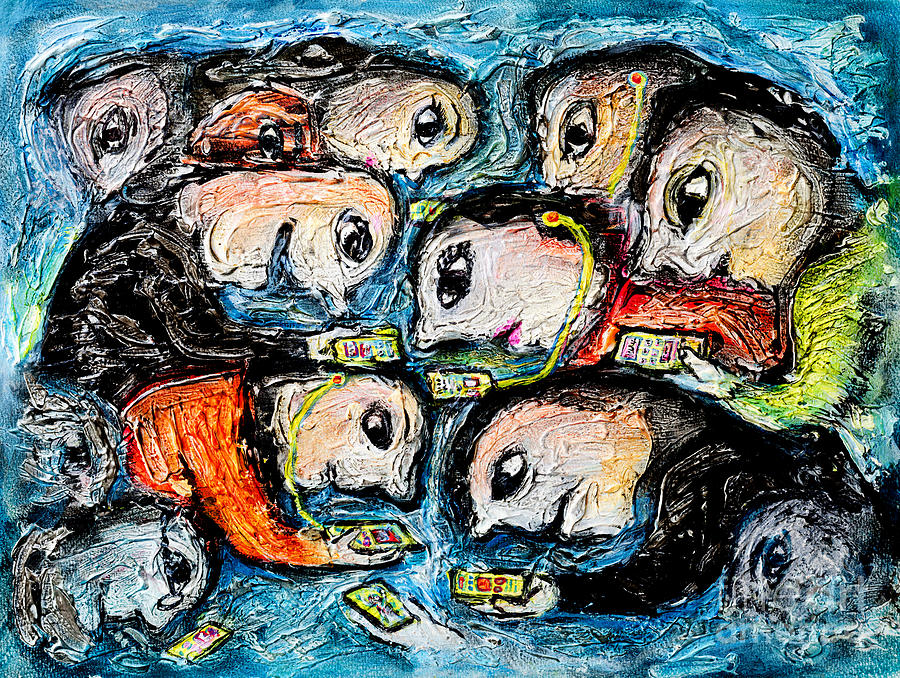The image is a detailed, abstract painting showcasing eleven distorted faces, each with exaggerated features like large eyes, pointy noses, and small ears. These faces are part of full upper bodies dressed in simple, colorful clothing, such as orange, yellow, and black shirts. All the figures are facing sideways, with those on the left turned towards the right and vice versa, and their heads are all tilted downward. Each person holds a phone, which emits a bright yellow light, emphasizing their apparent addiction to the devices. Some figures also have yellow earbuds with a reddish-orange center connected to their phones. The background is a swirl of blue and white, giving a watery, immersive feel, with the faces towards the corners fading into the blue, further enhancing the abstract and surreal quality. The painting's thick strokes add texture, making the depiction of the characters and their fixation on their phones more vivid and thought-provoking.